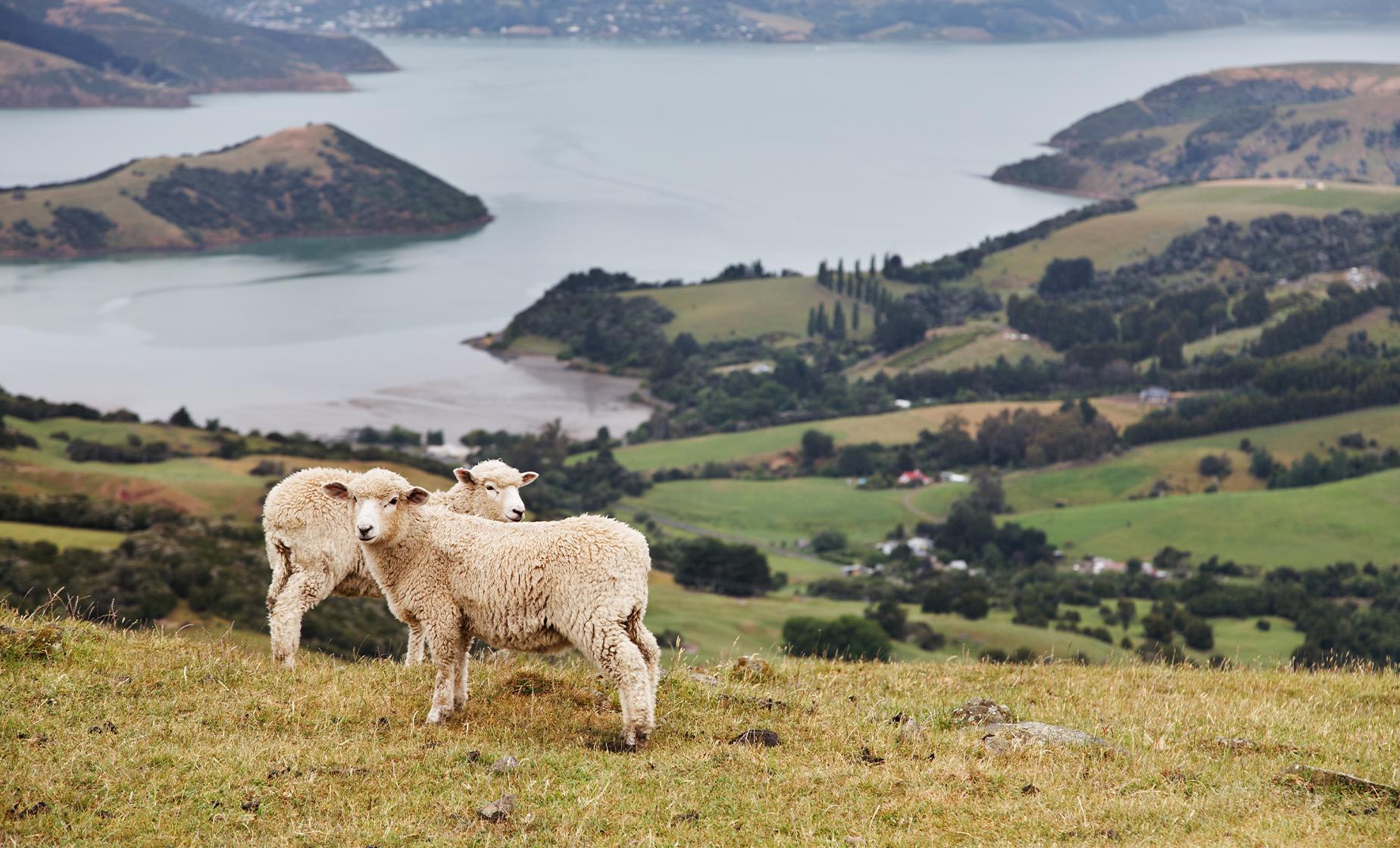A picturesque landscape stretches out before us, featuring a vast expanse of land dotted with rocks and covered in both yellow and green grass. Two white lambs with a slight hint of black and pink inside their ears stand on a grassy hillside in the foreground, gazing curiously at the camera. The field they're on is level and opens up to sprawling green fields below, interspersed with a few farmhouses. One farmhouse to the right boasts a red roof and white siding.

The background reveals a large, serene body of blue water, potentially an ocean inlet or bay, with a cone-shaped island situated in the center. Tree-covered mountains and grassy hills frame the water, some of which extend into the distance, leading one's gaze to a small, blurry town on the far side of the water. The scene is free of any text, allowing the natural beauty of the open field and its diverse elements to shine through.